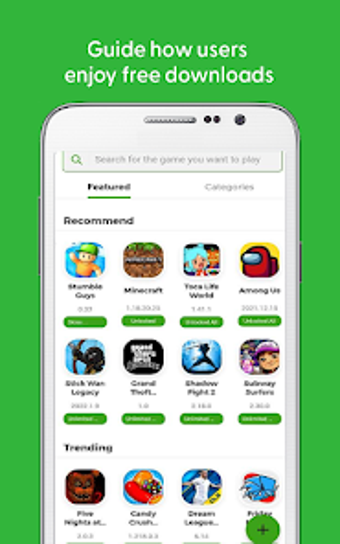The image is a promotional screenshot for a mobile application feature. The background is a bright green color, creating a vibrant and attention-grabbing backdrop. At the top center of the screenshot, there is a title in white, sans-serif, title-case letters with only the first letter of each word capitalized. The title reads: "Guide How Users Enjoy Free Downloads."

Below this title, there is an image of a phone, resembling an iPhone, portrayed as a template to showcase the app's features. The phone, depicted in white with a silver outline, has smoothly curved edges with approximately a 10-degree radius. At the top center of the phone, there is a long oval slit, likely representing a speaker or microphone, accompanied by two smaller circles and another circle, indicative of sensors and a camera.

The attention is focused on the phone's screen, which displays the app's interface. The screen features a white background with an assortment of app icons. At the top, there are two tabs: "Featured" on the left, highlighted with black text and a green underline, and "Categories" on the right, in light gray text, indicating it is not selected. Below the tabs is a section labeled "Recommended," presenting twelve app icons arranged in three rows and four columns.

The apps displayed include recognizable names such as Minecraft, Among Us, and Candy Crush. Each app icon is accompanied by text beneath it, along with green buttons, presumably indicating options to download or get more information about the apps.

The composition of the screenshot effectively highlights the app's feature for promoting free downloads through a well-organized and visually appealing layout.